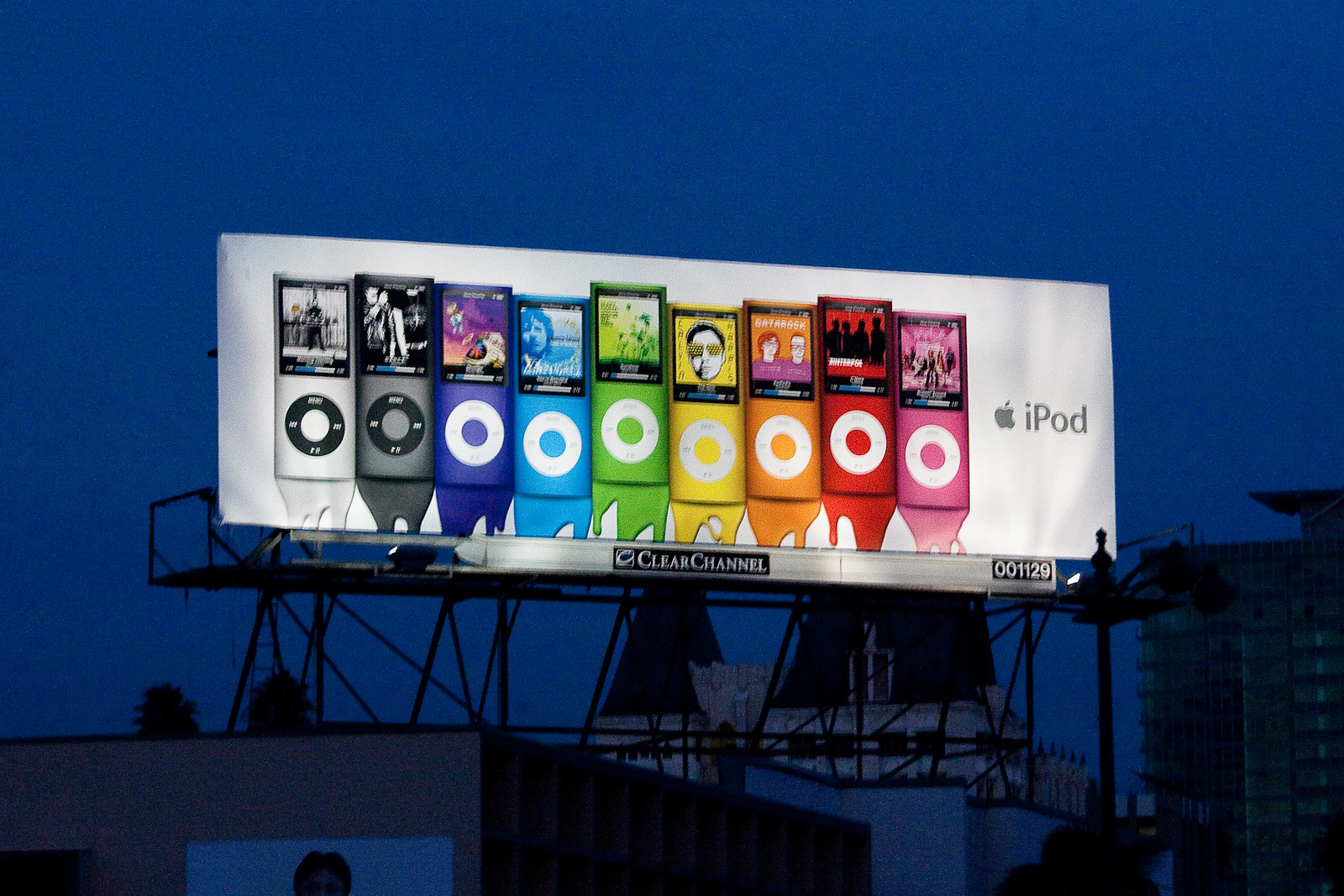This vibrant, color photograph captures a large, brilliantly illuminated billboard mounted on an intricate scaffolding structure amidst a bustling cityscape. The billboard, an advertisement for various iPod models, stands out vividly against the dusky, blue evening sky, suggesting that the sun has already set. Surrounding the billboard are numerous tall buildings, with a more historic, architecturally distinct structure visible in the background, just behind the ad.

The illuminated billboard showcases a striking array of iPods, each presented in a unique color. The arrangement starts with silver and black models, followed by a spectrum of rainbow hues. Each iPod screen displays a distinct design, adding to the visual appeal of the advertisement. The iPod logo is prominently positioned to the right of the colorful display. Below and to the right of the billboard, shadowy outlines of buildings add depth to the scene, emphasizing the height and prominence of the billboard within the urban landscape.